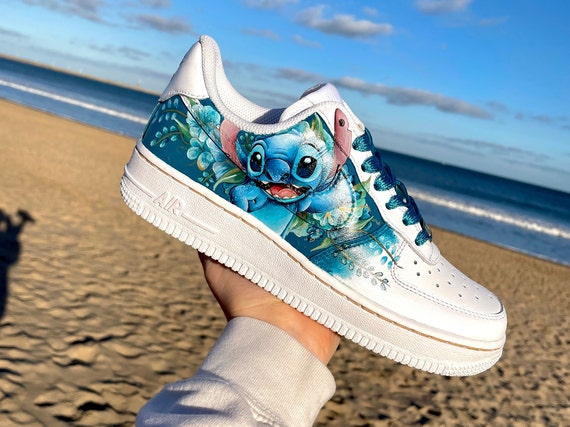A photograph captures a sandy beach setting with a blue sea lined with white waves and a sky adorned with white and grey clouds. The camera is tilted about 40 degrees to the right. In the foreground, a left hand, clad in a long-sleeved white T-shirt, holds up a white sneaker prominently featuring a painted design. The sneaker, notably marked with the word "AIR" near the heel, showcases an elaborate illustration of Stitch, the blue alien character from Disney's Lilo & Stitch. The detailed painting on the sneaker includes Stitch with big black eyes, a red tongue, open mouth, and pink floppy ears, alongside bursting blue flowers and green floral accents. The photograph’s composition also includes the subtle shadow of the person’s hand on the left, adding depth to the vivid beach landscape.